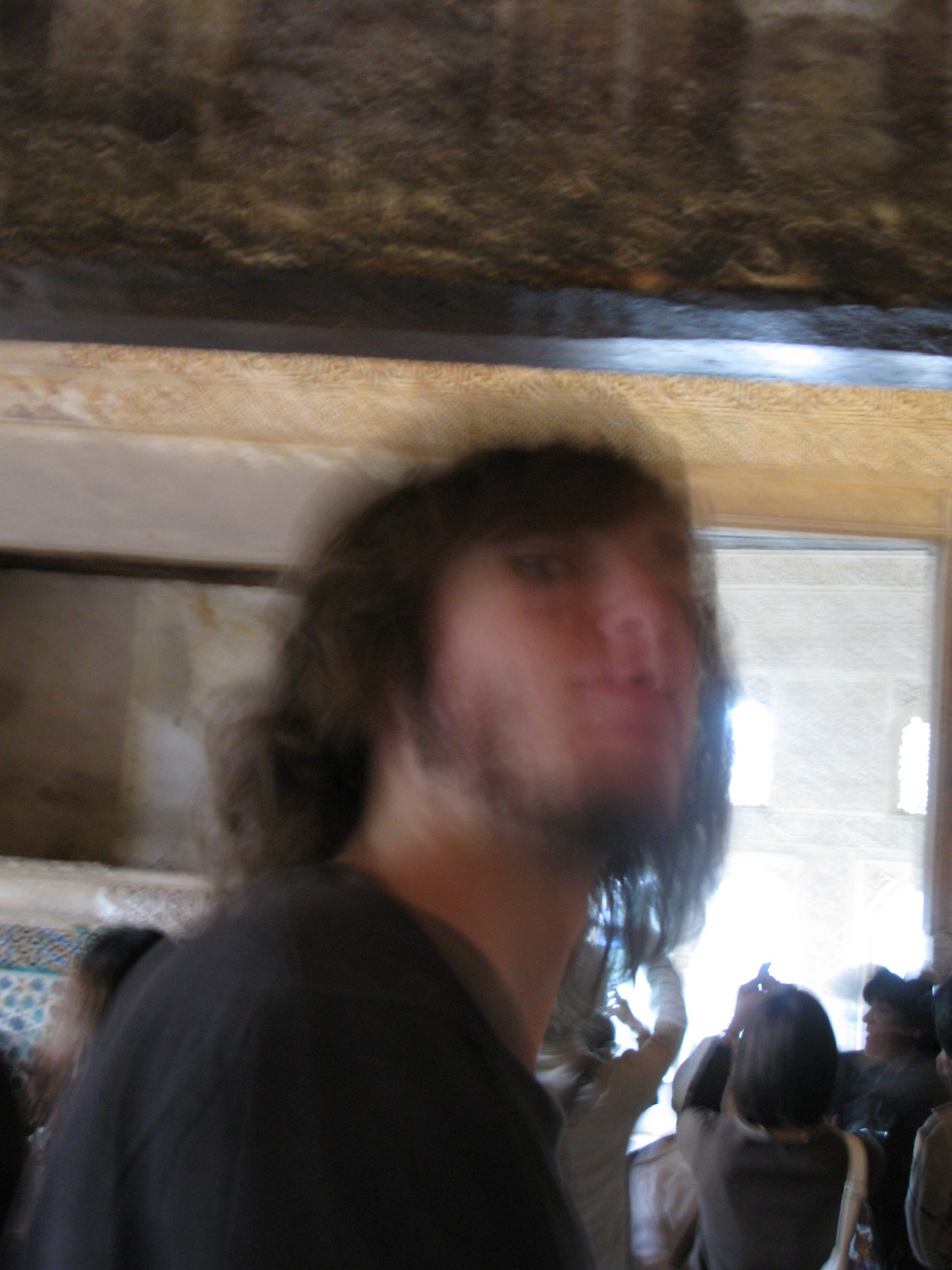The photograph depicts a blurry image of a young Caucasian male with medium-length, shaggy brown hair that touches his shoulders. He has scraggly facial hair, including a beard, and he is wearing a black t-shirt with obscured sleeves. The man's head is turned towards the camera, seemingly caught in motion, indicating he was not ready for the picture. Behind him, the background features a natural stone wall or ornate structure, with other details possibly indicative of a museum or historical site. Several individuals, presumably women, are visible in the background. They appear to be taking pictures or looking upwards, possibly at a ceiling or a display, suggesting they are on a tour. The setting is potentially a noteworthy or historical location in Europe, with visible elements like tiles and a possibly carved or brown ceiling. The overall image is very out of focus, making it difficult to capture finer details.